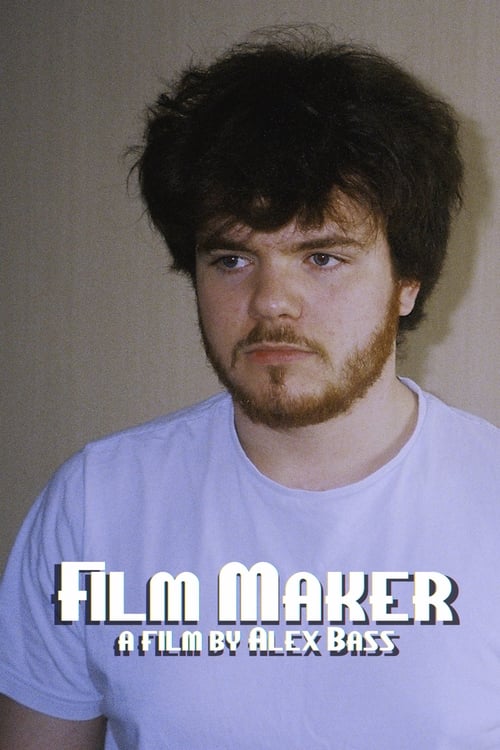This image features a man in his 30s facing towards the camera, though his gaze is slightly off to his right. His medium-length, bushy brown hair and a well-kept, closely-cropped beard, along with a thin mustache, frame his face. He has blue eyes and brown eyebrows. The man is dressed in a plain white t-shirt and is standing against a plain beige wall. The image captures him from the chest up, with his left arm out of the frame and only a small part of his right arm visible on the left side of the image. At the bottom of the photograph, white text with a black shadow reads "Filmmaker," with the words "A film by Alex Voss" below it in smaller white letters.